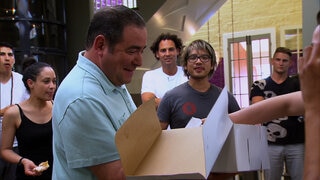The image captures a vibrant indoor scene centered around a middle-aged man of European descent, wearing a light blue shirt and sporting closely cropped black hair. He stands at the forefront, smiling warmly as he peers into a box that likely contains a cake or dessert. His joyful expression sets the welcoming tone. In front of him, a man extends his right hand into the box, contributing to the excitement.

Grouped behind the central figure are six casually dressed individuals. To the left, a woman in a black tank top smiles and looks off into the distance. Directly behind the man, a gentleman with glasses beams at the camera. Beside him, another man also smiles, enhancing the cheerful atmosphere. A man to the right, wearing a black V-neck shirt adorned with white skulls and jeans, stands with his arms crossed and gazes away thoughtfully. Additionally, two individuals in white shirts are partially visible in the background, adding to the overall convivial vibe. The scene appears to be celebratory, possibly on the set of a reality TV show, capturing a moment of shared happiness and camaraderie.